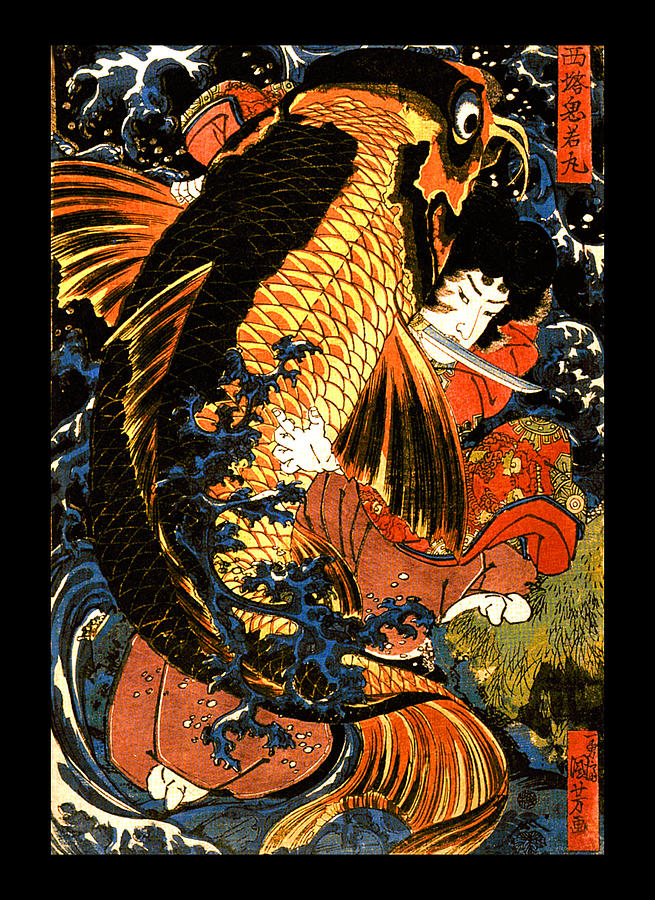This illustration, framed with a black border, brilliantly combines vibrant colors and intricate details. At its heart, the image features a colossal, multicolored bird and a vividly detailed fish, set against a dark blue and black background. The bird, predominantly black and yellow with striking orange streaks, perches atop a person whose white face and black hair are partially visible. The fish, with exaggerated features such as large eyes, fins, and scales, appears in shades of orange, gold, yellow, white, and tinges of blue, resembling a catfish. Adding to the rich tapestry of elements, an Asian language vertically adorns an orange banner on the top right, and possibly the sides, complementing the scene. Additionally, a man with long hair, Asian features, and clad in a red kimono wielding a sword, emerges from the composition, enhancing the complex narrative of the artwork.